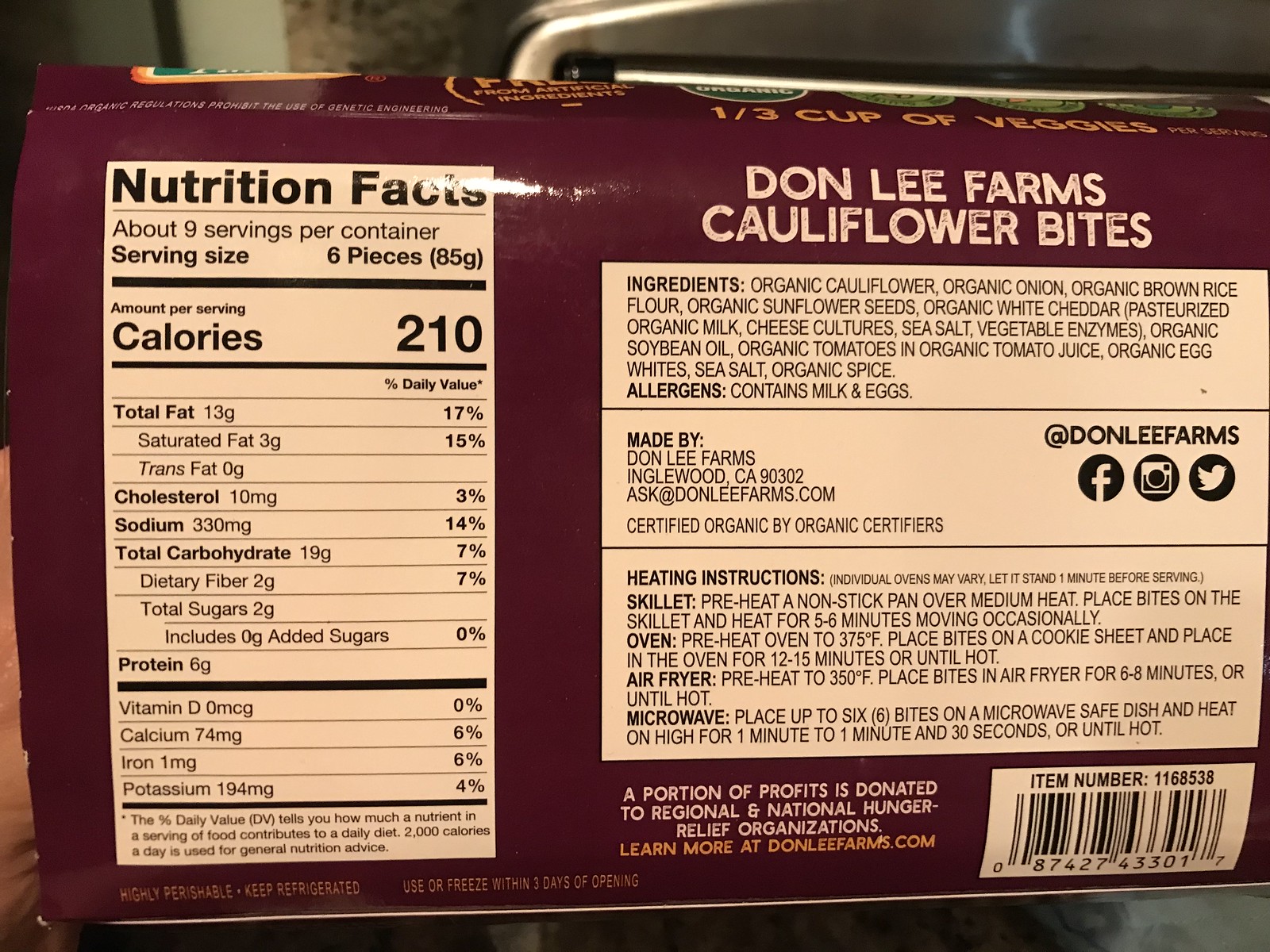The image features a package of Don Lee Farms Cauliflower Bites set against a background of indistinct silver metal and some brown and white hues. The package itself is a vibrant purple with bold white lettering that reads "Don Lee Farms Cauliflower Bites." Displayed prominently are the nutritional facts, indicating that the package contains about nine servings, with a serving size of six pieces. Each serving provides 210 calories.

The nutritional information is clearly printed in black text on a white background and includes: 13 grams of total fat, 3 grams of saturated fat, 0 grams of trans fat, 10 milligrams of cholesterol, 330 milligrams of sodium, 19 grams of carbohydrates, 2 grams of dietary fiber, 2 grams of total sugars (with no added sugars), and 6 grams of protein. Additionally, it lists vitamin D at 0%, 74 milligrams of calcium, 1 milligram of iron, and 194 milligrams of potassium. Beside these values, the daily percentage values are also provided.

The package notes that the product is made by Don Lee Farms, located in Inglewood, California, 90302. The company can be contacted via their website at donleefarms.com. The product is certified organic by Organic Certifiers and includes heating instructions along with a detailed ingredient list. Allergen information indicates that the product contains milk and eggs.